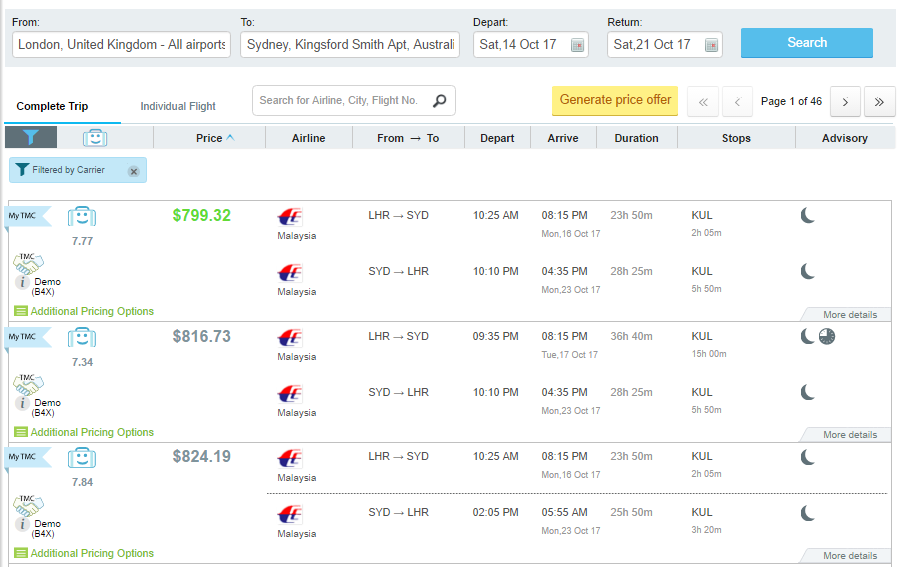A detailed screenshot of a travel website displaying flight options for a round trip from London, United Kingdom (all airports) to Sydney, Kingsford Smith Airport, Australia. The departure date is set for Saturday, October 14, 2017, with a return date of Saturday, October 21, 2017. Although the website's name is not visible, this is not Google Flights. The user has selected "Complete Trip Flights," with the cheapest option priced at $799.32. This particular flight, operated by Malaysian Air, departs from London Heathrow (LHR) at 2:25 AM and arrives in Sydney (SYD) at 8:15 PM, totaling a duration of 23 hours and 50 minutes, including a 2-hour layover. The flight has a moon symbol advisory, indicating it is a night flight. Two additional flight options are listed below, also operated by Malaysian Air, priced at $816.73 and $824.19 respectively.